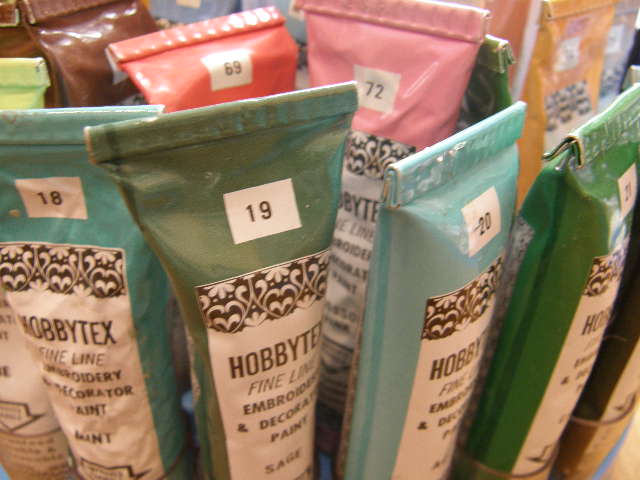This slightly out-of-focus photograph, likely taken by a cell phone, showcases an array of colorful tubes of paint arranged closely together, clearly displayed on a store shelf. Each tube is uniformly designed, reflecting the color contained within—ranging from multiple shades of green (including mint and sage) to light blue, olive green, brown, bright green, red, pink, and orange. Prominently featured on the front of each tube is a white rectangle adorned with a black and white scrolled detail at the top, beneath which reads "Hobbitex Fine Line Embroidery and Decorator Paint." Numbers such as 18, 19, 20, 21, 69, and 72 are visibly marked within these rectangles, which also display the name of each specific color, like "mint" and "sage." The tubes collectively brandish a consistent layout, reinforcing that they are all products from the same Hobbitex line.